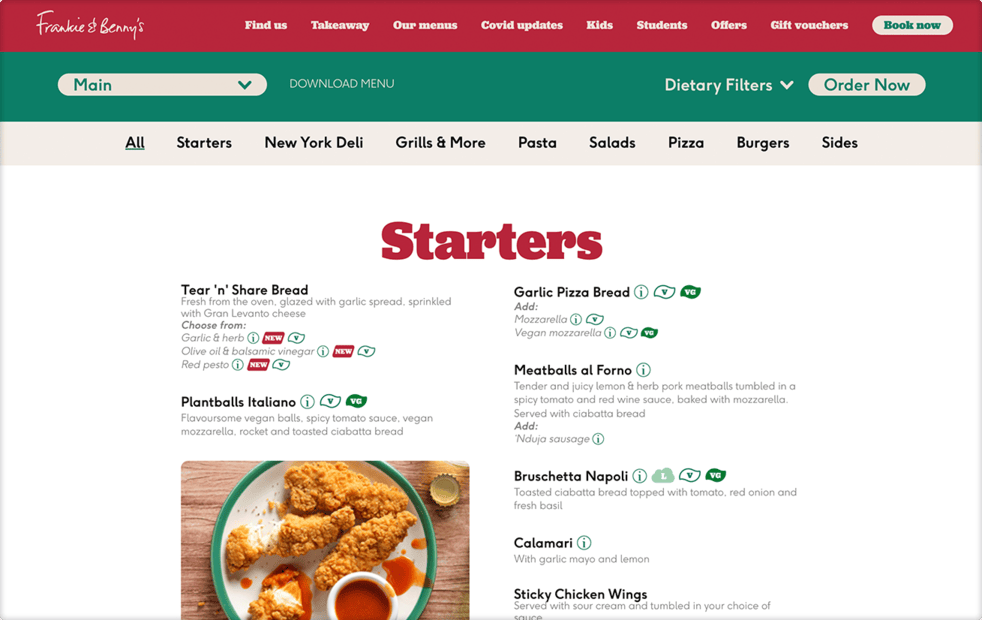This image is a detailed screenshot of Frankie and Benny's restaurant website. The layout begins with a prominent red header that features the restaurant's name, "Frankie and Benny's," written in an elegant cursive font at the left. Moving rightward, there is a sequence of white serifed text links for navigation, offering options such as "Find Us," "Take Away," "Our Menus," "COVID Updates," "Kids," "Students," "Offers," and "Gift Vouchers." In the top right corner, a distinctive white pill-shaped button with teal text reads "Book Now."

Beneath this red header, a teal secondary header appears. On the left, it includes a white pill-shaped dropdown menu labeled "Main" with a teal arrow indicating further options. Adjacent to this, outside the menu area, a white all-caps link "Download Menu" is displayed. Further along to the right, another prominent white text link "Dietary Filters" is coupled with a downward-facing white arrow. Finally, at the far right, another white pill-shaped button with teal text invites users to "Order Now."

Directly below the teal header, a light gray strip spans the width of the page, featuring navigational links in black text. The links, encompassing "All," "Starters," "New York Deli," "Grills and More," "Pasta," "Salads," "Pizza," "Burgers," and "Sides," are punctuated by the teal-underlined "All" to indicate the current selection.

The body of the webpage features a clean white background with the menu content. Centered at the top is the category heading "Starters" in large red text. Below, menu items are meticulously arranged in two columns. Each item begins with a bolded black title. For example, the top-left item is "Tear and Share Bread," followed by a detailed description in smaller, light gray text: "Fresh from the Oven Glazed with Garlic Spread Sprinkled with Gran Levante Cheese." This structured format continues consistently throughout the menu.